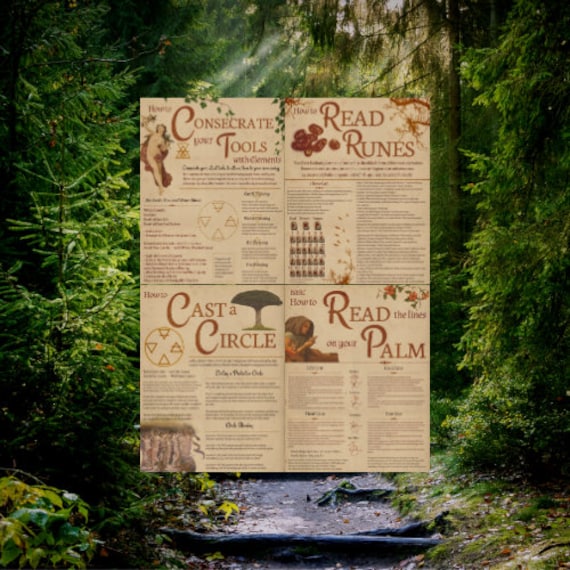The image shows a tranquil forest setting, with sunlight filtering through tall trees, illuminating a serene stream flowing over moss-covered rocks and surrounded by foliage. Overlaying this picturesque scene is a large rectangular arrangement of four pages from a book or poster, placed in a two-by-two grid. These pages offer detailed how-to guides on mystical practices. The top left page, titled "Consecrate Tools," features an illustration of a cherub. The top right page is labeled "Read Runes" and contains various runic symbols. The bottom left page, titled "Read Palm," provides information on interpreting the lines on one's palm. Lastly, the bottom right page, "Cast a Circle," includes an image of a tree and a circle with triangular symbols. Intricate writing accompanies each section, though the text appears somewhat blurry. The backdrop of lush trees and the sparkling river enhances the mystical, almost enchanted feel of this composite image.